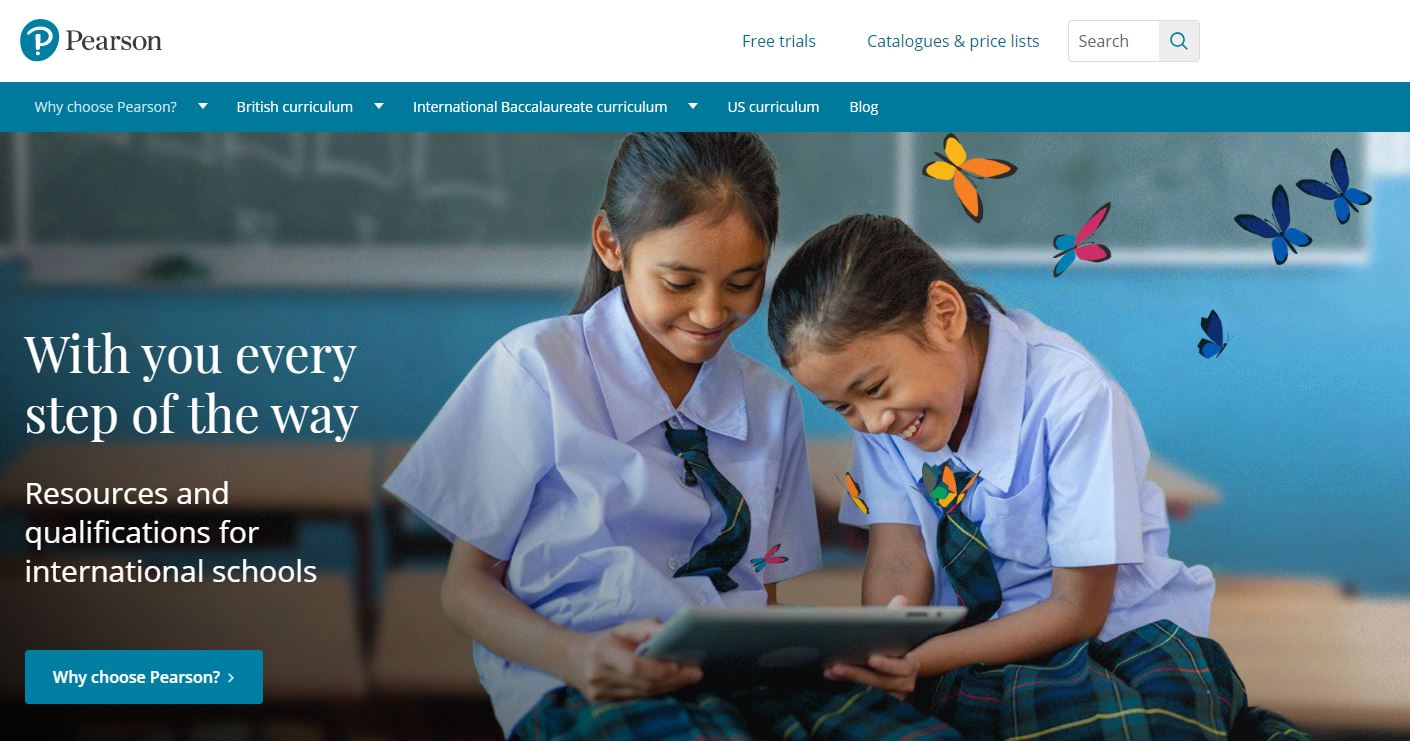This image, sourced from the Pearson website, artfully captures two young girls in school uniforms, enthusiastically engaging with a tablet. The girls, dressed in plaid skirts with matching ties and blue shirts, sit at a desk in a classroom with blue-green walls. They smile brightly, suggesting they could be playing a game or exploring educational content on the tablet. Surrounding them are additional desks, contributing to the academic atmosphere.

At the top of the image, a blue-green banner harmonizes with the classroom's color scheme, featuring text that highlights Pearson's educational offerings: "Why choose Pearson" alongside options for the Irish/British Curriculum, International Baccalaureate Curriculum, U.S. Curriculum, and a blog. Additional navigation options include free trials, a catalog, a price list, and a search area.

Decorative butterflies adorn the right side of the image, adding a playful touch. The compelling tagline reads, "With you every step of the way—resources and qualifications for international schools." Below this, a teal button reiterates the invitation with the prompt, "Why choose Pearson." This meticulously crafted image underscores Pearson's commitment to providing comprehensive educational resources globally.